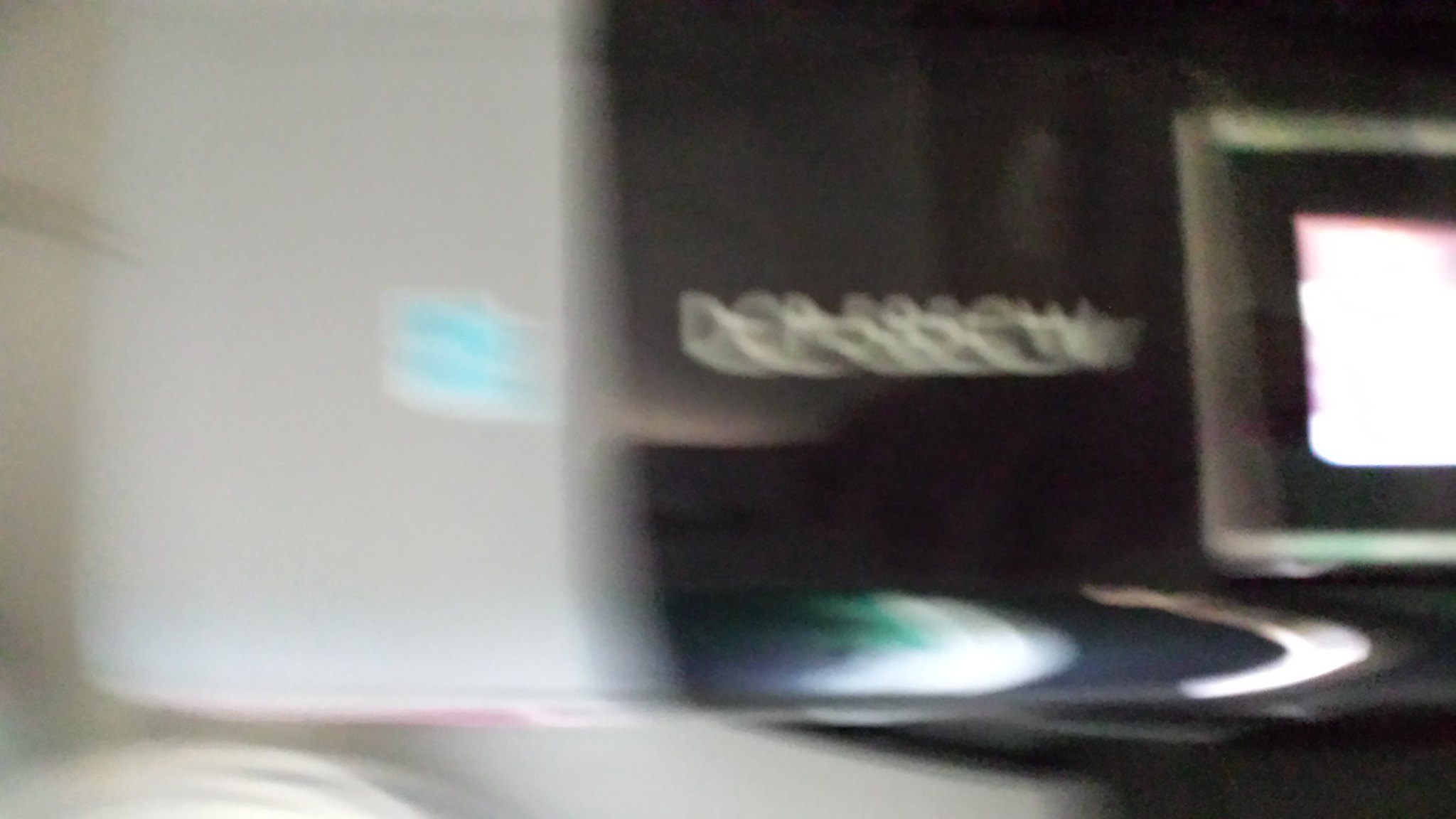In this very blurred horizontal image, the scene appears to be a close-up of desk items. On the right side, there is a computer monitor with a silver frame displaying a bright, indiscernible rectangular image. Adjacent to the monitor, white text can be vaguely deciphered, potentially reading "DEP 585 CW" amidst an expanse of blurred white space. To the left side of the image, there's a large, possibly white-framed device, which might be another computer or a printer, featuring a noticeable blue square in the middle. In between these two main elements, there is a shiny black object that could be a brochure, CD, or black record. The overall color scheme of the image includes predominant whites and blacks with occasional hints of green and blue. The blurriness suggests the camera was moved during the capture, adding to the challenge of identifying the finer details.